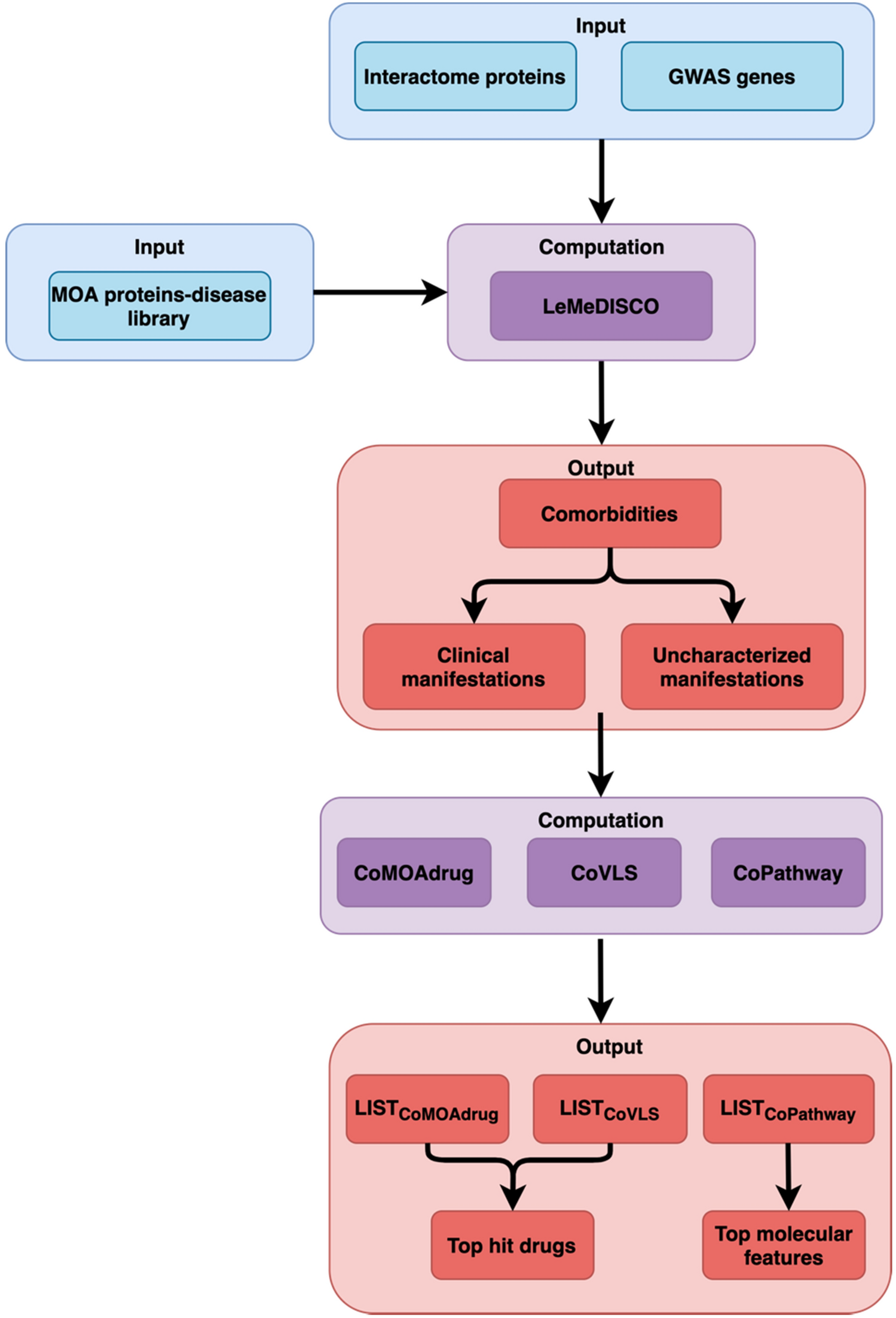This image depicts a scientifically detailed flowchart, likely generated by computer, featuring various interconnected rectangles and arrows. At the top, in a blue box labeled "Input," it lists "Interactome Proteins" on the left and "GWAS Genes" on the right. A black arrow leads downward to a purple rectangle labeled "Computation." To the left of this, another flowchart box, also titled "Input," includes a smaller blue box containing "MOA Protein-Disease Library," with a black arrow pointing rightward toward the "Computation" box. 

Beneath the "Computation" box, a red rectangle is connected by a downward arrow to another purple rectangle, and this is followed by another black arrow leading to an additional red rectangle. The overall flowchart consists of five main rectangles aligned vertically, interconnected by black, straight arrows, with another critical input source stemming from the independent left-sided box. The typography used is a standard, clean font such as Times New Roman or Arial, ensuring clarity in the depiction of the data flow. Despite detailing various categories and their connections, the flowchart does not include a title, leaving its specific purpose undefined.